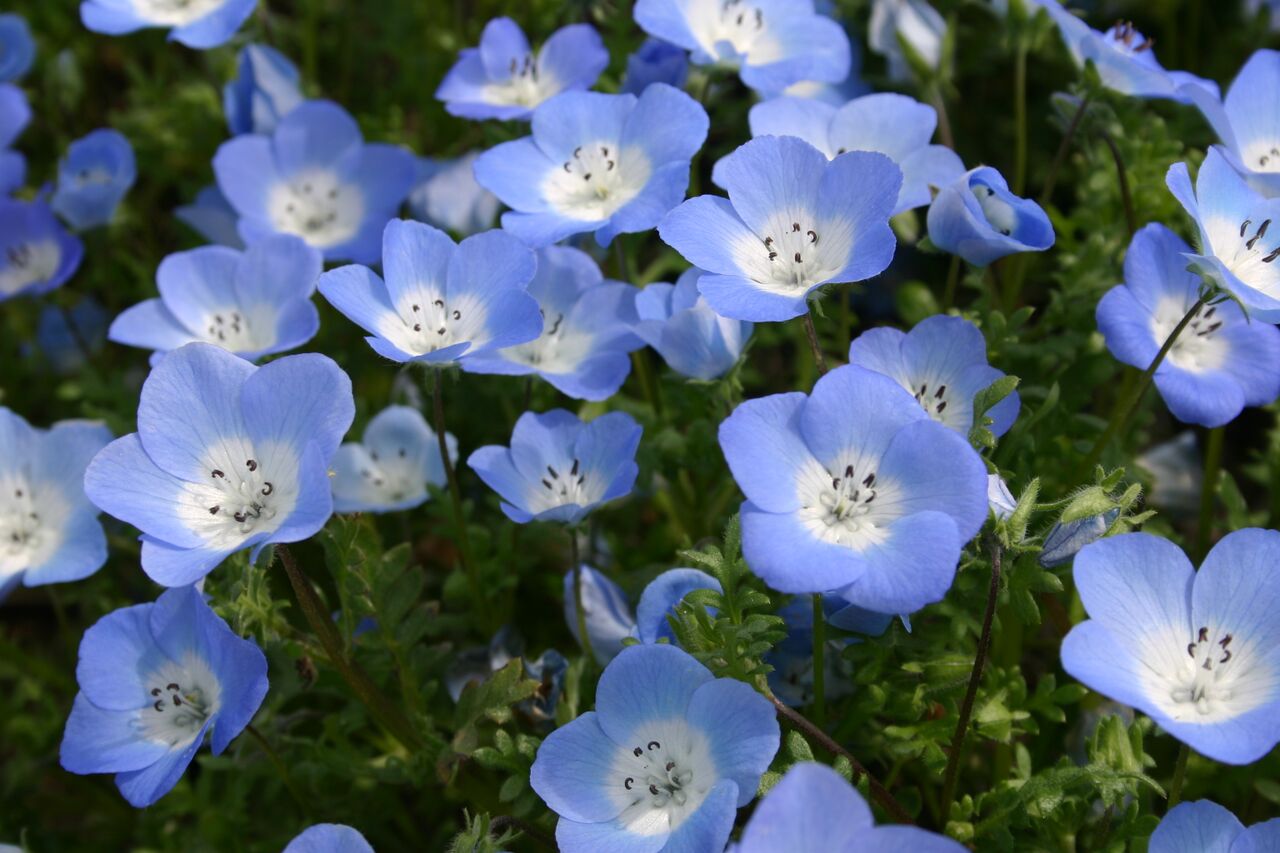This close-up image captures a vibrant field of delicate light blue flowers, each characterized by five petals and a central cluster of white stems with dark tips. The blossoms fill the upper left of the frame, appearing denser and more in focus there, while thinning out toward the bottom and right sides where some greenery and weeds are visible. The flowers are bathed in sunlight, which highlights their fine details and the various shades of green in the leaves and stems. Some flowers towards the back of the image are just beginning to bloom, their petal tips tinged with a deeper purple. The overall scene is a harmonious blend of blossoming flora and lush greenery.